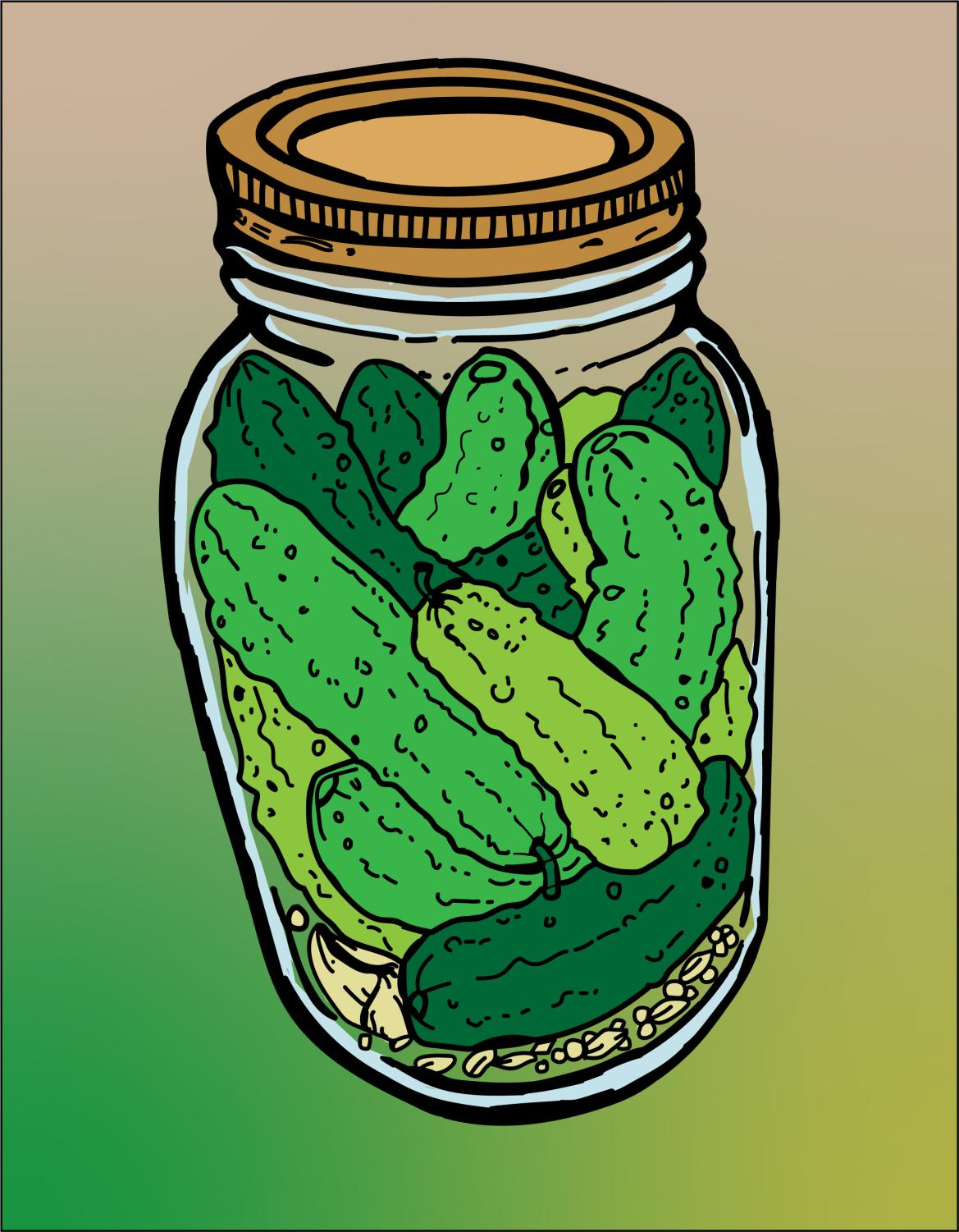This digital illustration features a quart-sized mason jar filled with green cucumbers, also referred to as pickles, in a variety of shades ranging from dark to medium to olive green. The jar, outlined with thick black lines in a cartoonish style, has a clear glass body highlighted with white accents and is sealed with a gold, screw-top lid adorned with a decorative edge. The background displays a gradient, starting with a light pinkish-tan hue at the top that fades into a medium green on the lower left and shifts to a pea soup green on the lower right. Inside the jar, which is drawn with meticulous black outlines, the pickles are textured with wrinkles and some have small green stems. The entire scene is framed by a thin black line border, adding a cohesive and detailed touch to the illustration.